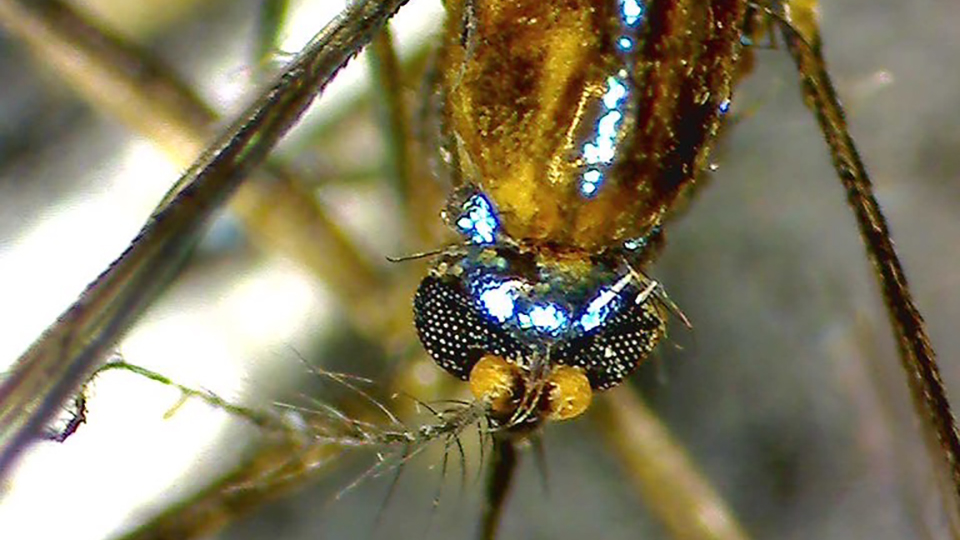This is a close-up photograph of an unidentified insect, viewed from the top. The insect's body is a shiny, irregularly shaped brown, with a glossy appearance on its abdomen. Its eyes are large, bulbous orbs that spread across its face, appearing black with fine net-like white dots. The eyes also have a hint of gold and blue. The mouthparts of the insect are yellow, contrasting with the brown of its abdomen. The legs are long, thin, and spread out to the sides, featuring fine, spiky hairs and displaying a brownish-green hue. The antennae are not prominent in this image. The background is out of focus, blending shades of gray, white, and brown.